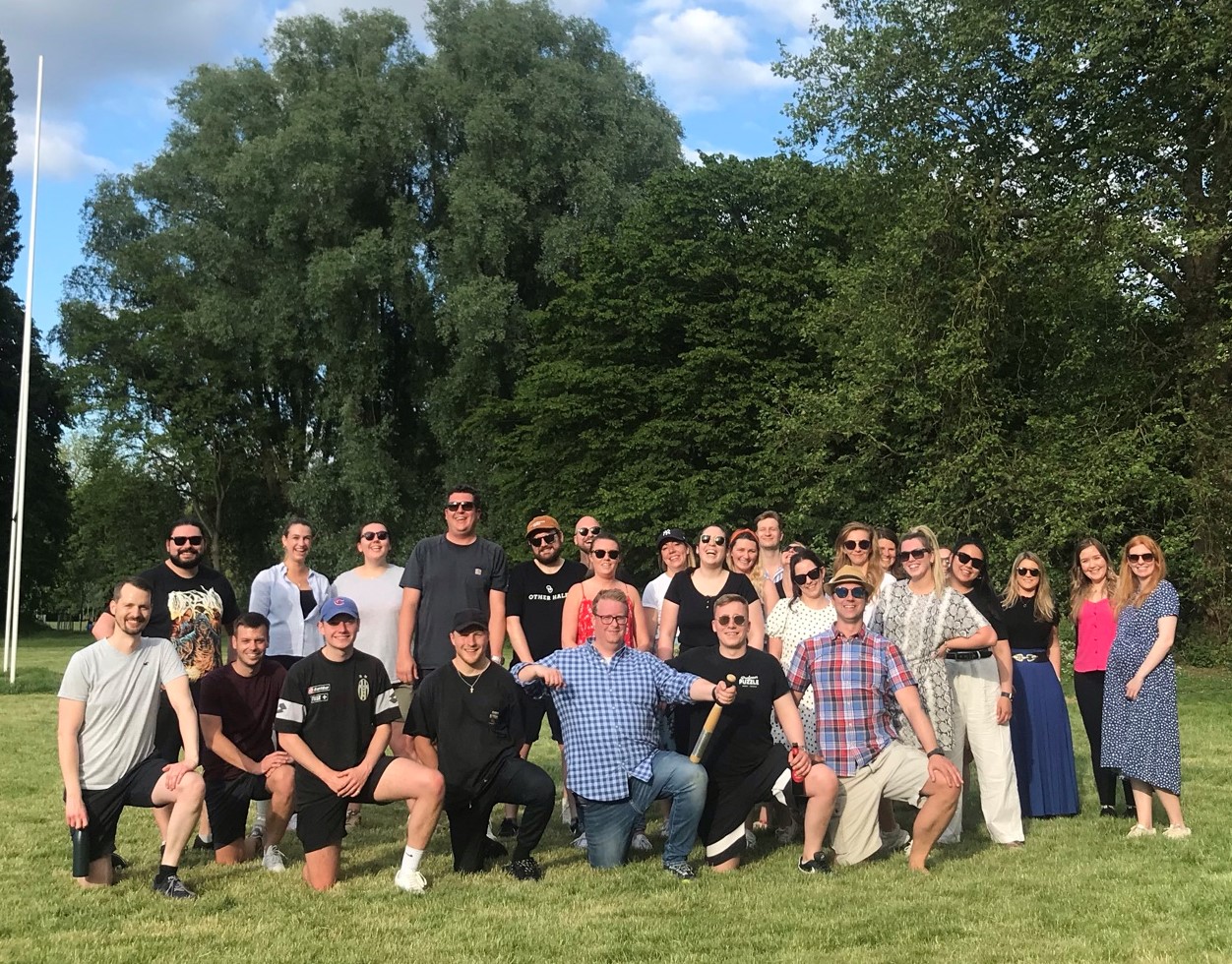The photograph captures a lively group of approximately 25 to 30 adults, predominantly in their 30s to 40s, posing for a group photo in an outdoor setting. They are arranged in three distinct rows on a lush green field—about seven men kneeling in the front row, their right knees on the ground and left knees up, while the rest of the group stands behind them in two lines. The group consists of a mix of men and women, with a noticeable array of black sunglasses shielding their eyes from the sunlight. They're dressed in casual, summer attire, including t-shirts, shorts, jeans, dresses, and skirts. 

The backdrop features three towering trees with abundant green foliage, and a blue sky with a smattering of white, fluffy clouds peeking through. A tall, white flagpole is visible on the left side of the image, extending high into the sky. Everyone is beaming, adding a joyful energy to the scene; a woman on the far right stands out with her vibrant orange hair and blue dress, suggestive of pregnancy. A man positioned centrally is notable for holding a brown bat with a gray end in his left hand, potentially indicating the occasion for the photo. It seems to be a captured moment of camaraderie, possibly within a park, underlining the shared happiness of the group's gathering.